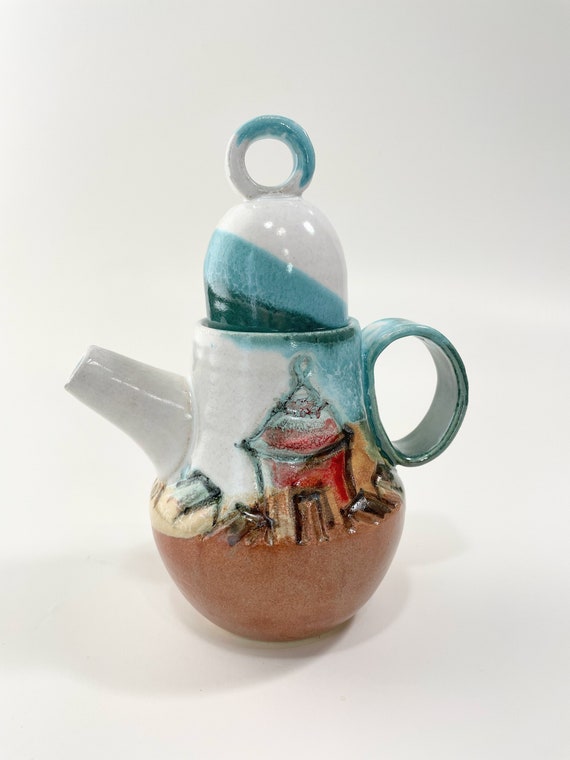The photograph is of a small, shiny, ceramic teapot set against a light gray background with a white area in the middle, placed on a white surface with a slight shadow beneath it. The teapot has a brown base, and as the eye moves upward, it features a carved artistic image depicting what looks like a small red hut with a brown door, flanked by a white area on the left and a light blue area on the right. The teapot has a standard handle on the right side that is turquoise in color, and a matching turquoise and white handle on the lid, which is loop-shaped. The lid itself is adorned with white, light blue, and dark blue stripes. The spout of the teapot is white. The entire piece is glossy, indicating a glazed finish, and despite the intricate design, the artistic detailing is somewhat blurry and not sharply defined. There are two sources of light that illuminate the teapot, enhancing its reflective ceramic surface.